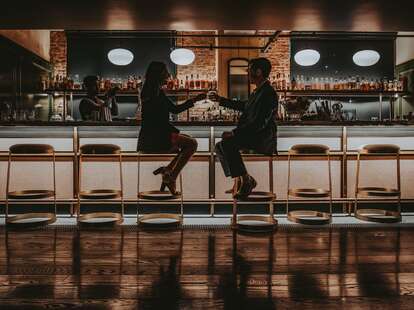This horizontal photograph, reminiscent of a movie still, captures an intimate, dimly lit bar scene set against a backdrop of red brick walls with white mortar. The bar area features two shelves filled with various bottles of alcohol and is illuminated by a combination of four bright white lights and several warm yellow lights that hang from a dark brown, reflective ceiling. The floor, made of shiny, dark brown wood, adds to the cozy ambiance.

A bartender stands in the shadows to the left of the scene. At the center of the image, a professionally dressed couple in their 20s or 30s is seated on black-topped, metal-framed bar stools, facing each other. The man is on the right, and the woman on the left, both partially obscured by shadows, clinking their glasses in a toast. This carefully arranged composition highlights the couple's interaction, adding to the photograph's atmospheric and intimate mood.